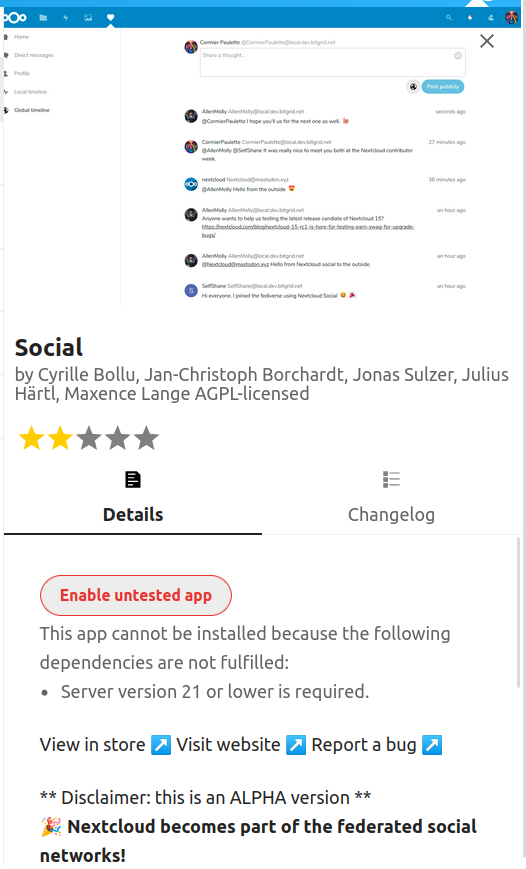A screenshot reveals a profile view of a web browser window displaying a social media platform interface. At the top, a header presents options to "Share a thought" and "Post," indicating it is a social media feed. Below the header, the word "Social" is prominently displayed in bold black text. 

The section beneath lists various contributors, including Cyril Bolu, Jan Kristoff Forged, Jonas Sulzer, Julius Hartl, Maxon Sling, and indicates the AGPL License. This is followed by a star rating system, where only two out of five stars are highlighted in yellow, suggesting a low rating.

Two toggle buttons are visible; "Details" is selected and emphasized in black, while "Changelog" is greyed out. A warning message in a red circular badge reads "Enable untested app." Additionally, a disclaimer states, "This app cannot be installed because the following dependencies are not fulfilled," accompanied by options to "Visit in store," "Visit website," and "Report bug."

The screenshot ends with a final note: "This is an alpha version," and a cautionary message implying, "This cloud becomes part of the federated social networks. Terrifying."